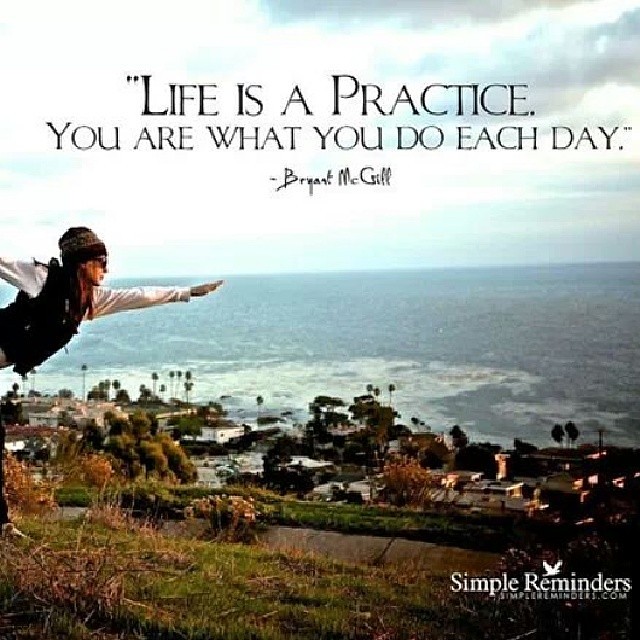A man stands poised on one leg at the top of a hillside overlooking a serene shoreline that meets the expansive ocean stretching to the horizon. He wears a vest over a long-sleeve white shirt, a beanie cap, and sunglasses. His arms are outstretched front and back, appearing to balance gracefully. The sky above is partly cloudy, casting a soft light over the scenic landscape. Text overlaying the image reads, "Life is a practice. You are what you do each day," attributed to Bryant McGill. In the bottom right corner, a logo reads "Simple Reminders."